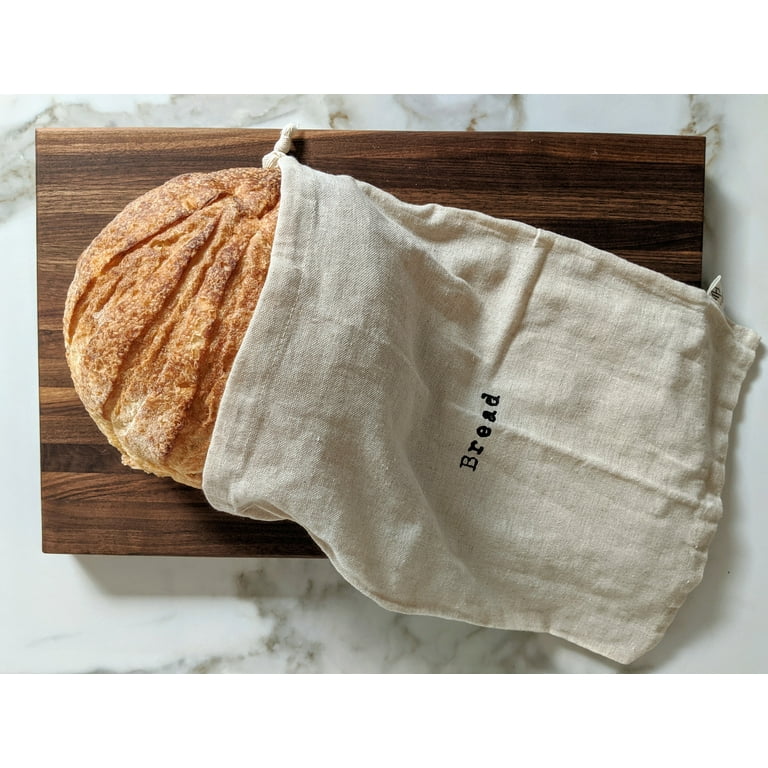The photograph depicts a rustic, round loaf of artisan bread, half of which is nestled inside a cream-colored linen bag. The loaf itself is positioned to the left side of the image, displaying a gradient of light to dark brown crust with distinctive cut marks on the top, indicating it was homemade. The linen bag, positioned at the center of the image, features the word "BREAD" prominently written in black font and is loosely tied at the top into a knot to the right. The bag rests on a rectangular dark brown wooden cutting board, showcasing visible wood grain patterns. This cutting board is placed on a marble countertop with an off-white base interspersed with light gray and black veining, indicating the indoor kitchen setting of the photograph. The overall composition emphasizes the rustic and homey atmosphere of artisanal baking.